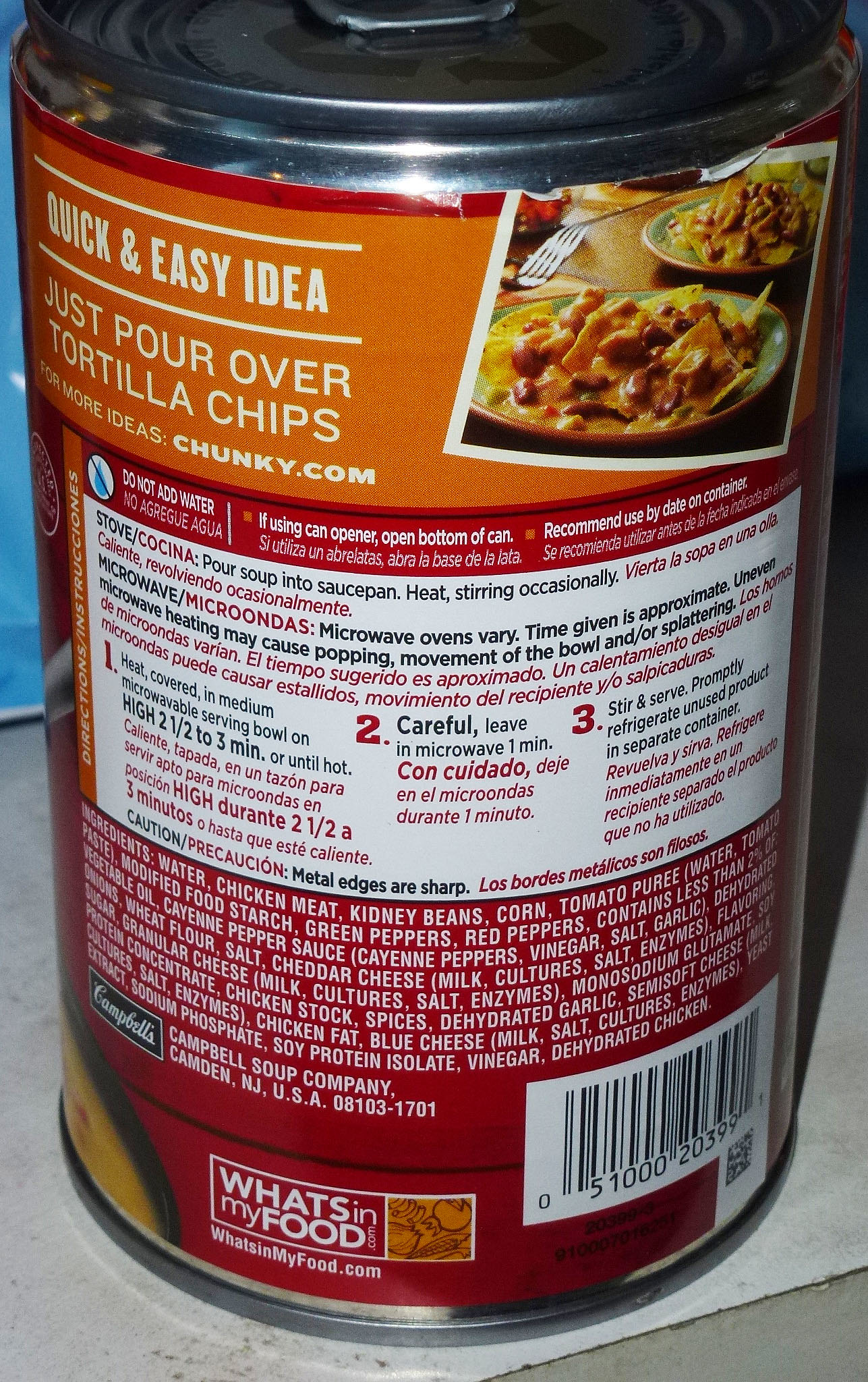The image prominently features a circular can, occupying the majority of the frame and set against a white platform. The can is topped with a silver lid and adorned with a detailed label. In the upper left corner of the label, the text reads: "Quick and easy idea. Just pour over tortilla chips. For more ideas: chunky.com." To the right of this text, there is a vivid illustration of two plates filled with brown beans and tortilla chips. Beside these plates, a spoon and a fork are placed, suggesting a ready-to-eat, convenient meal.